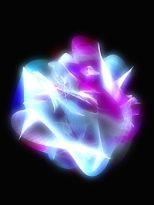The image is an abstract, organic, and fluid-like digital artwork rendered against a solid black background. It features a mass of swirling colors including white, pink, blue, and hints of turquoise. This mass appears to be floating in space, with varying degrees of clarity: some areas appear blurry with a fog-like effect, while others have well-defined lines creating a sense of movement. Lighting appears to highlight specific sections of the mass, casting certain areas in bright light which then fade into darkness, creating a dynamic interplay of light and shadow. The color scheme is predominantly purplish-pink towards the center, with white and blue elements swirling around the edges, and additional purplish-pink tones towards the bottom left. The overall effect is reminiscent of a long-exposure photograph capturing the trails of neon lights, presenting an ethereal and nebulous visual experience.